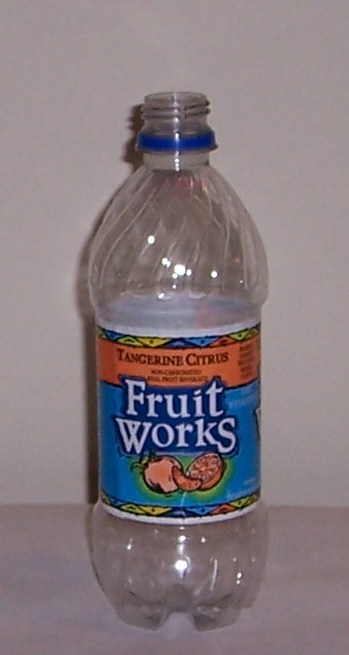In the rectangular photograph, a clear, empty bottle, which could be either plastic or glass, stands on a cream-colored shelf or table. The bottle lacks a cap and is shaped like a typical single-serving soda bottle. The bottle features a colorful label: the top part of the label has a pink background with the text "Tangerine Tangerine Citrus" in white. Below that, against a blue background, the text "Fruit Works" is displayed in white letters, and at the bottom, images of an orange and a banana are visible. The wall behind the bottle is a grayish-white color, providing a neutral backdrop that contrasts with the vibrant label of the bottle.